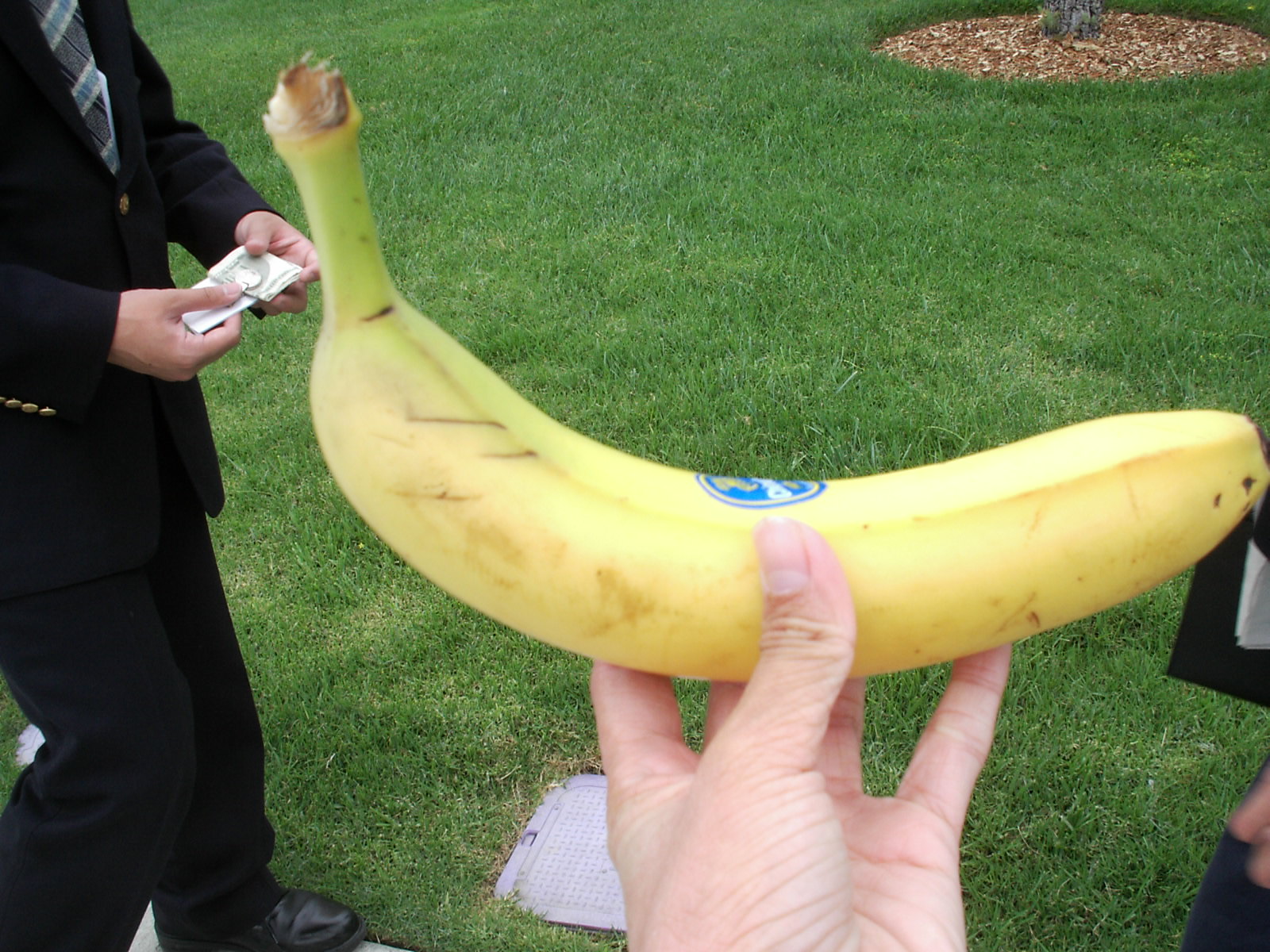In this image, a man prominently holds up a single, perfectly ripened banana. The banana features a few small brown spots, which appear more like scuff marks, while its stem remains green, indicating its freshness. The photograph's background reveals another man dressed in a dark blue suit, who is looking down, seemingly at a rectangular object such as a card or lighter. He is also wearing polished black leather shoes and stands on a paved path adjacent to a grassy area. Behind him, a tree trunk surrounded by mulch is partially visible. In the immediate vicinity of the person holding the banana, a plastic utility tub is situated beneath his hand. Additionally, there is a glimpse of another formally dressed individual on the right side of the image, discernible by a portion of their suit and a slightly blurred hand. The entire focus of the photograph is on the banana, and all individuals in the image have light skin tones.